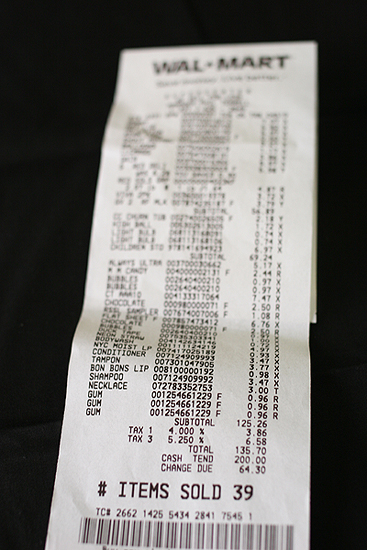This photograph depicts a crumpled Walmart receipt against a black background, possibly a sheet. The receipt itself is quite wrinkled and out of focus, particularly in the upper half where the text is mostly obscured by blurred lines. Despite the poor quality of the image, the bottom portion reveals the last eight purchased items: NYC Moist, Conditioner, Tampon, Bon Bons, Shampoo, Necklace, and three entries for Gum. The subtotal for these items is $126.26, and after tax, the total amounts to $135.70. There was a cash payment of $200, resulting in a change of $64.30. The receipt indicates that 39 items were sold in total, and it features a barcode at the bottom.